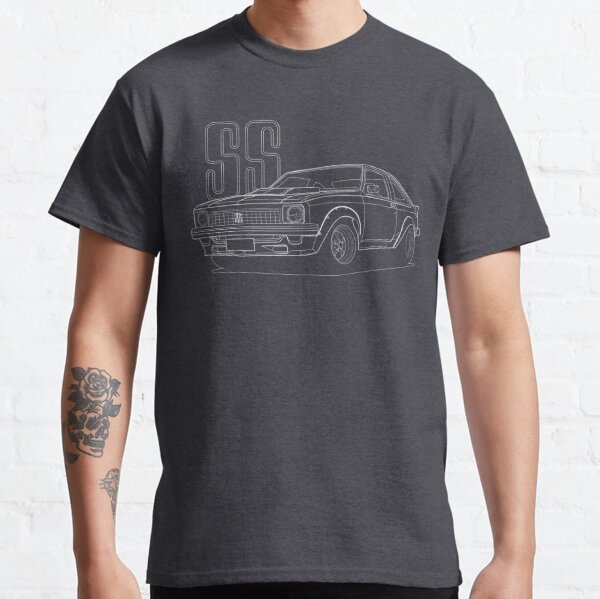The image depicts the torso of a pale white male model, estimated to be between 17 and 22 years old, showcasing a gray crewneck t-shirt. The photograph is framed from just above his neck down to his waist, with his arms resting at his sides. The t-shirt features a detailed outline of a two-door sports car with sporty wheels, likely a Ford Mustang, with the designation "SS" for Super Sport prominent near the upper left of the car. The car's hood is raised, suggesting a high-performance engine beneath. The male model's left forearm is adorned with a striking tattoo of a skull entwined with a rose, while another indiscernible tattoo is visible closer to his wrist. He pairs the t-shirt with black pants, only a sliver of which is visible in the shot. The background consists of a white brick wall, providing a contrasting backdrop to the model's gray attire.